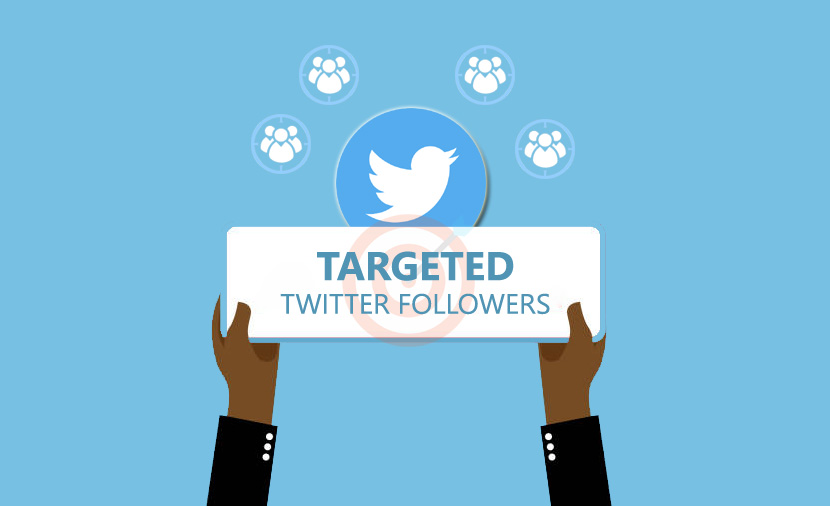The screenshot displays a website dedicated to selling targeted Twitter followers. The background of the page is light blue, giving it a calm and professional appearance. Positioned at the top center is the iconic Twitter logo, which is a dark blue circle featuring the well-known white Twitter bird.

Flanking this logo are four circles, two on each side. These circles each contain profile images of people, likely representing users or testimonials. 

Beneath the Twitter logo is a prominent white text box. Inside, bold text reads "Targeted Twitter Followers." Lightly superimposed in orange within the text is a bullseye, emphasizing precision and targeted growth.

Supporting the text are two illustrated black hands emerging from either side of the box, as if holding it up. These hands wear black long-sleeve shirts adorned with three white buttons on each cuff.

Overall, the design is clean and straightforward, focusing on the service offered without any additional distractions or text.